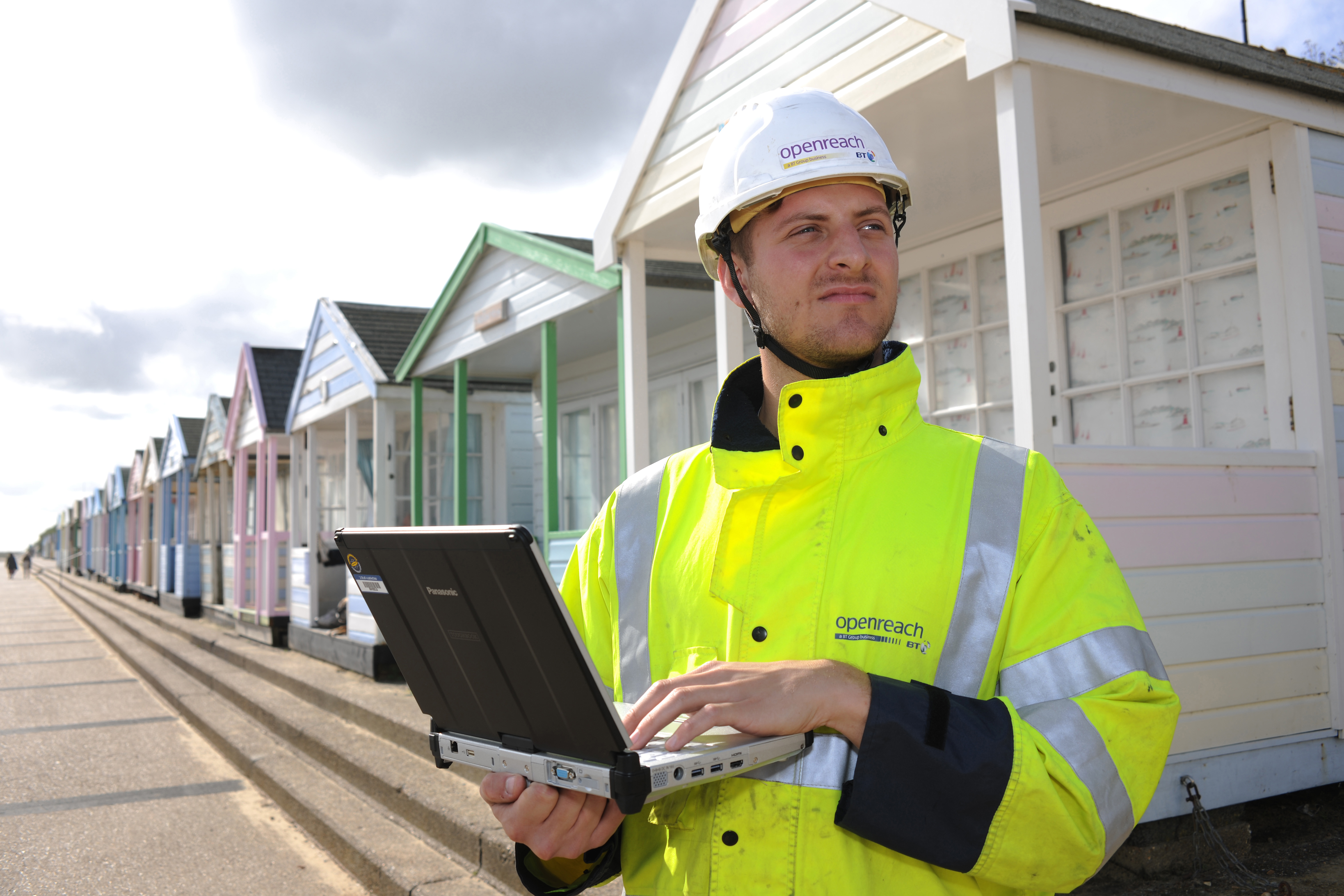In this outdoor daytime photograph, a white man wearing a fluorescent green jacket with reflective gray tape and a white construction helmet is the focal point. Both his jacket and helmet are branded with the word "Open Reach." He holds a laptop computer in his hands and gazes upward, slightly away from the camera, perhaps in contemplation or assessment. The backdrop features a row of small, identically styled houses, each with a porch, a gabled roof, and distinct trim colors including white, green, blue, and pink. Blue, beige, and pink accents adorn these homes, enhancing their quaint charm. To the side, you can see two individuals walking in the distance, adding life to the scene. A set of three steps lead up to each house. The sky overhead is overcast, casting a diffused light over the entire setting, contributing to the thoughtful and professional atmosphere of the image.